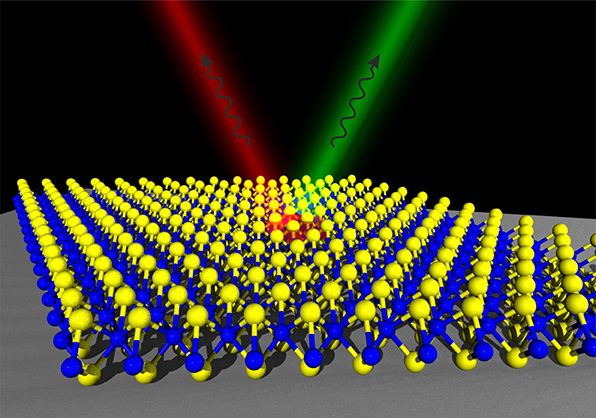In this computer-generated image, a meticulously organized arrangement evokes the classic children's game of jacks. Rows upon rows of stylized jacks, their spherical ends alternately colored in blue and yellow, extend into the distance, creating a pattern reminiscent of DNA strands. The jacks are positioned with precision on a gray, flat surface, their symmetry and repetition creating a sense of infinite continuity. A stark black background accentuates the foreground's vibrant colors. Cutting through this orderly scene, two diagonal spotlights intersect at the center: one emitting a red beam and the other a fluorescent green. Within these beams, squiggly lines with arrowheads point upwards, adding dynamic elements to the otherwise orderly composition. Each spotlight's contrasting color and shape dramatically emphasizes the structured yet colorful array of jacks below.